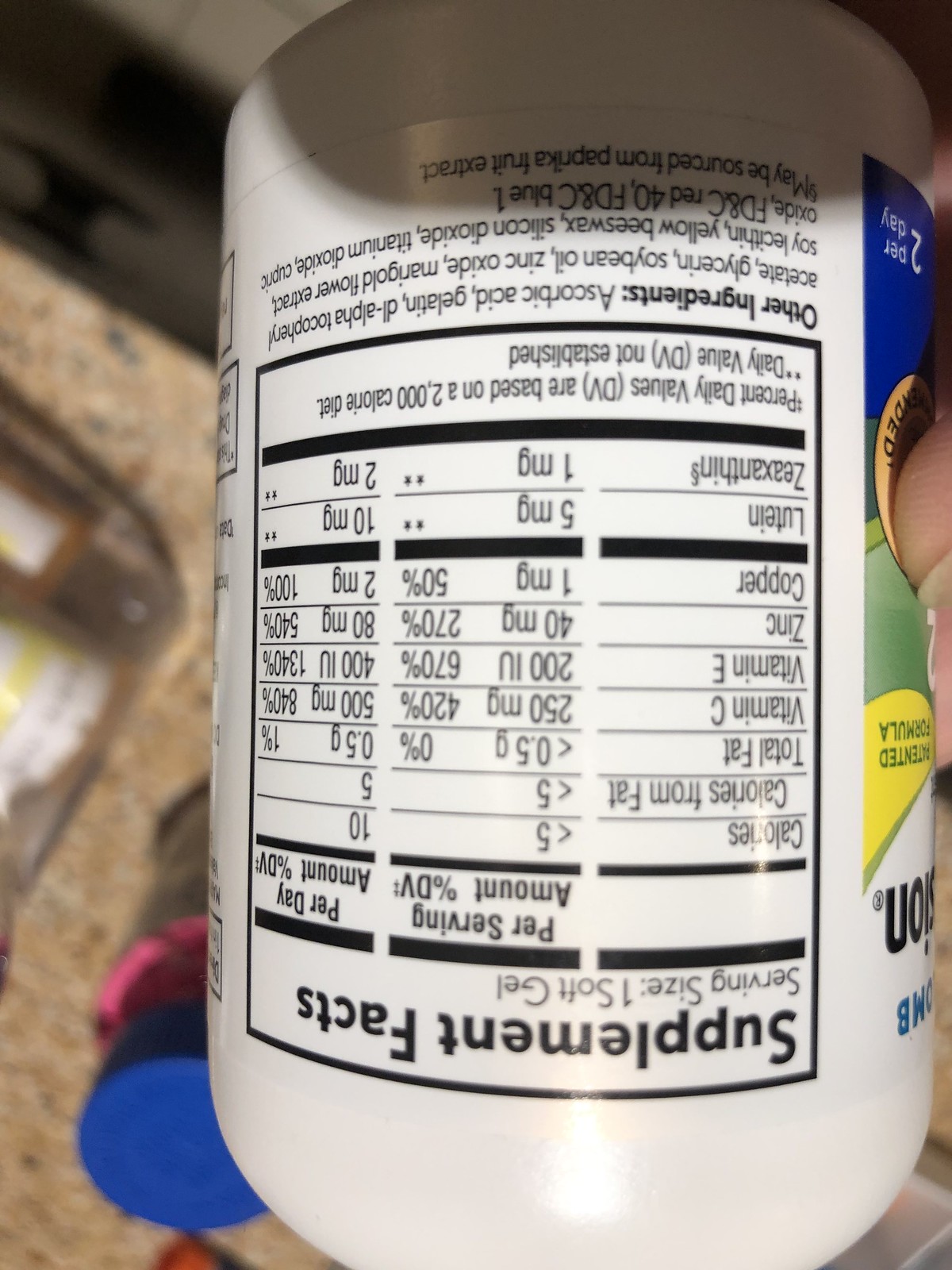The image shows an upside-down photo of a white vitamin bottle being held, with its blue cap removed and placed alongside a small pot of vitamin tablets on a granite countertop. The focus is on the Supplement Facts label, which lists the serving size as one soft gel. The label details the calories, how much come from fat, and the quantities of vitamins C and E, zinc, and copper per serving. It also notes other ingredients like ascorbic acid and gelatin. Although the brand name isn't visible, the text is black, with some portions in darker fonts. The label features a mix of green, blue, pink, and yellow colors. In the background, orange pill bottles with white labels are partially visible, indicating a collection of various medicines and dietary supplements.